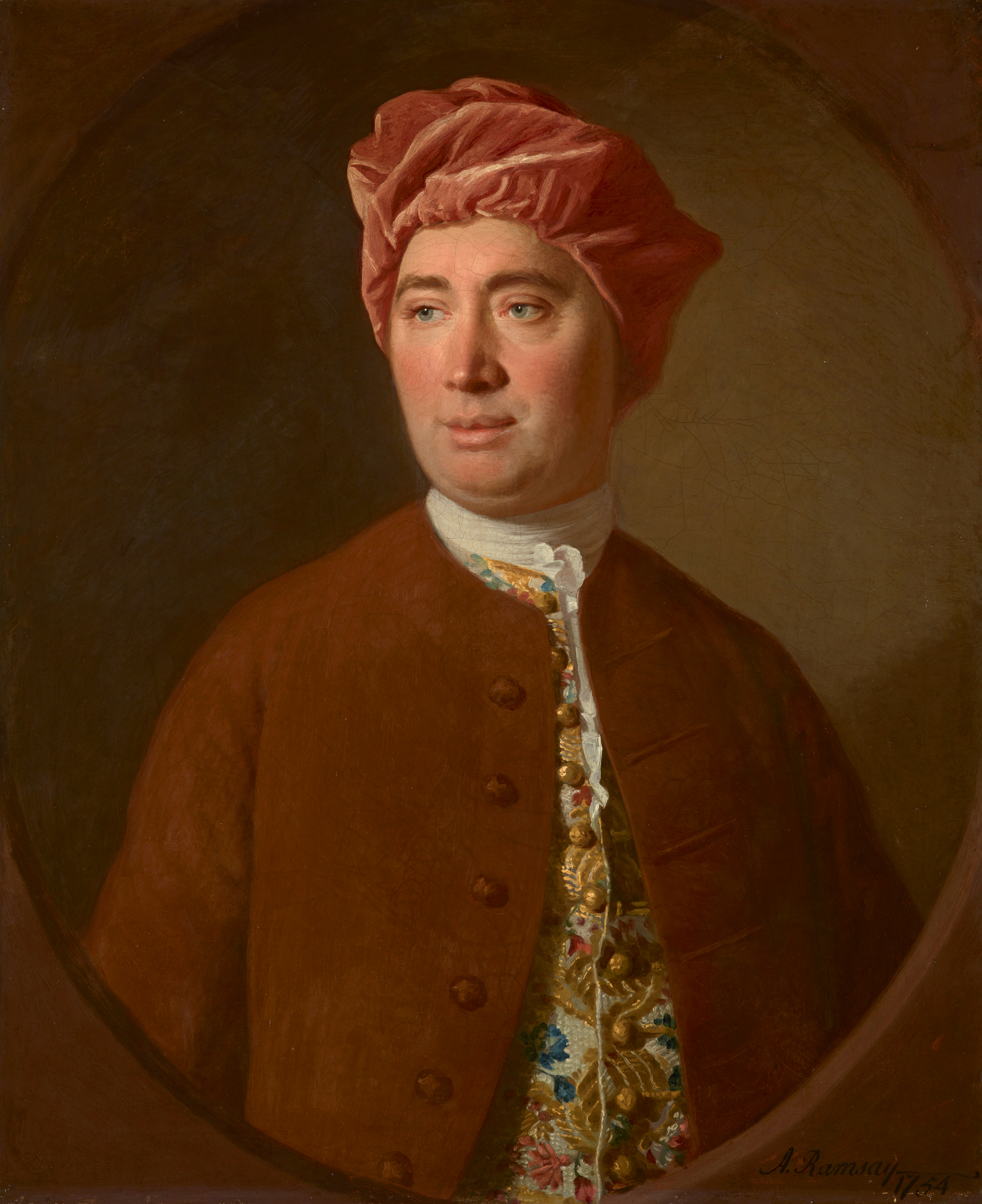This detailed caption describes an 18th-century portrait:

In this intricate 1754 portrait by A. Rumsey, a man is depicted in a striking ensemble reflecting the exotic Eastern styles that became fashionable in the 18th century. Atop the man's head is a rose-colored velvet turban hat, known as an "Ala Turk," which was often worn at home as a stylish alternative to a wig. The man exudes a stoic demeanor, with his gaze directed thoughtfully to the left.

The man's attire complements the exotic theme, featuring a burnt orange jacket layered over an ornate shirt adorned with numerous buttons and vibrant colors, including yellow, green, and red. The shirt boasts elaborate patterns and a prominent white collar that stands out against the rich hues of his jacket. 

The portrait is presented within a circular frame, accentuating the timeless quality of the image. The year "1754" is inscribed on the frame, providing historical context to this exquisite capture of 18th-century fashion and aesthetic sensibilities.